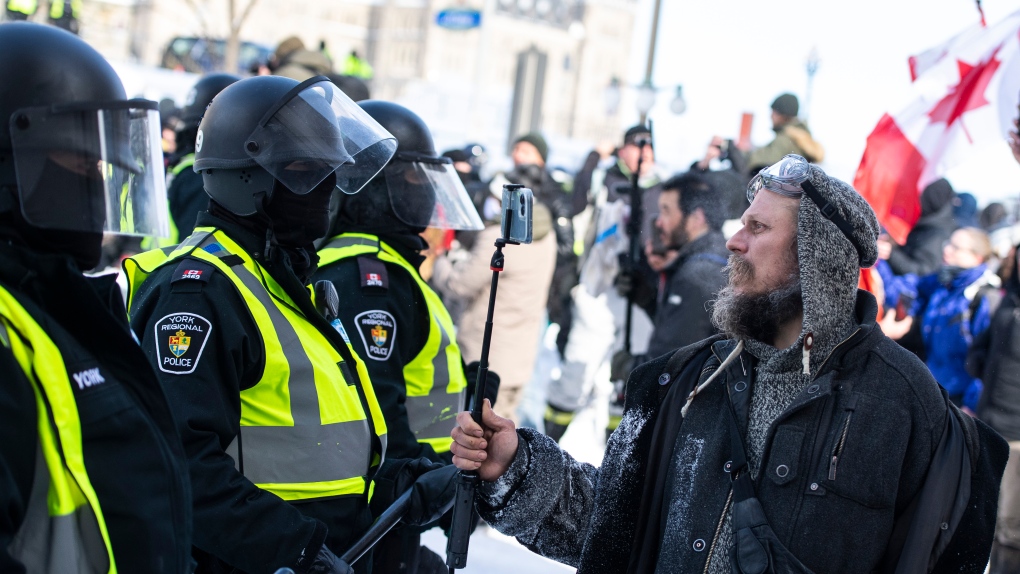The photograph captures a tense moment at a protest, evident from the standoff between several York Regional Police officers and a bearded, middle-aged protester. The officers, three of whom are distinctly visible and facing the right side of the frame, are clad in full riot gear, complete with helmets, face masks, and yellow reflective vests. The identification "York Residential" is visible on the sleeve of one officer's right arm. The protester, dressed in dark winter clothing with a hood and goggles resting on his forehead, is holding a cell phone on a selfie stick pointed directly at the middle officer. Behind him, the scene is filled with other demonstrators, most of whom are also dressed in dark attire, although a few breaks in the monotony appear, such as a woman in a royal blue coat and another individual in a tan coat. Canadian flags are prominently visible, suggesting the location of the protest is in Canada. The blurred cityscape in the background doesn't provide many geographical clues, but the late afternoon light implies the action is escalating as day turns to evening. Despite the palpable tension, the encounter appears non-violent, characterized more by a silent standoff than by chaos.